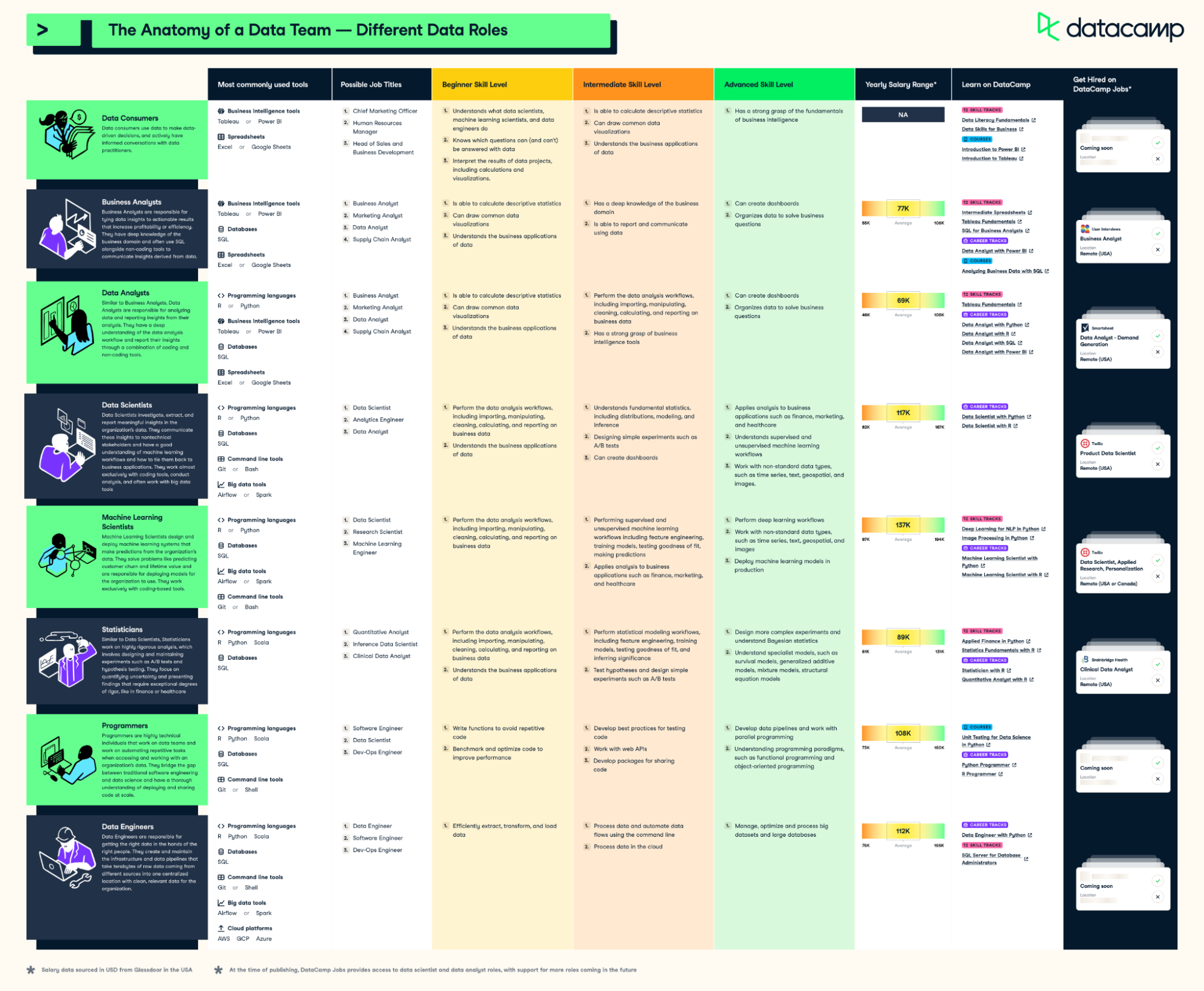This image features an intricate, multi-color print design primarily organized into a grid layout of eight rows and eight columns. The top portion of the graphic includes a green banner with blue text stating "The Anatomy of a Data Team - the Different Roles," positioned to the left, and a black "Datacamp" logo accompanied by a small DC icon in green at the top right. The entire right side of the image resembles a column of white rectangles that appear like envelopes, each containing small, unreadable text. The left side consists of alternating blue and green boxes filled with text and illustrations explaining various roles within a data team, such as data consumers, business analysts, data scientists, machine learning scientists, and data engineers. Despite the details provided, the small size of the text makes it difficult to read specific descriptions or titles accurately.